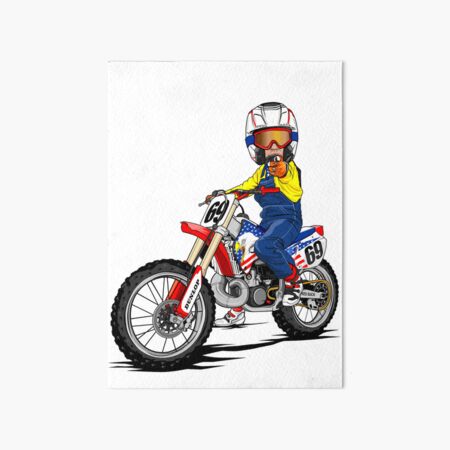The image depicts a cartoonish art print of a person riding a dirt bike against a white or off-white, slightly speckled with gray background. The bike appears to be themed around American symbols, adorned with a red, white, and blue flag and an eagle design. The bike prominently features the number 69 on both the front and backside. The tires are large, black, and chunky with visible spokes. The rider is wearing blue overalls and a yellow long-sleeved shirt, with orange gloves. They are pointing directly at the viewer, holding what appears to be a metallic object. Their right hand grips the handlebar while their left hand points outwards. The rider dons a mostly white helmet with red and blue stripes, and gold-tinted goggles framed in red. The bike also features light gold and red bars and "Dunlop" branding on the fork area.